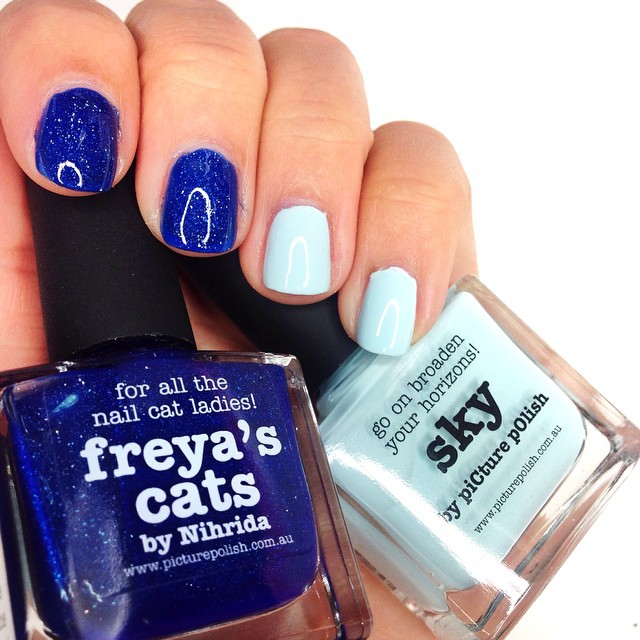The image shows a close-up of a woman's hand, showcasing an elegant manicure. Her index and middle fingers are adorned with dark blue nail polish infused with glitter, while her ring and pinky fingers are painted in a very light, almost whitish blue color. Each of her nails features meticulous detailing, adding a touch of sophistication. In her grasp, she holds two bottles of nail polish corresponding to the colors on her nails. The blue bottle, labeled "For All the Nail Cat Ladies, Freya's Cats by Picture Polish," stands out with white print against its rich blue background. The light blue bottle is labeled "Go On, Broaden Your Horizons, Sky by Picture Polish," carrying the message in a similarly elegant font. Both bottles share black caps and sit snugly in her palm, their labels clearly visible, suggesting that this visually appealing image is likely a social media advertisement for the nail polish brand or a promotional post by a fashion influencer.